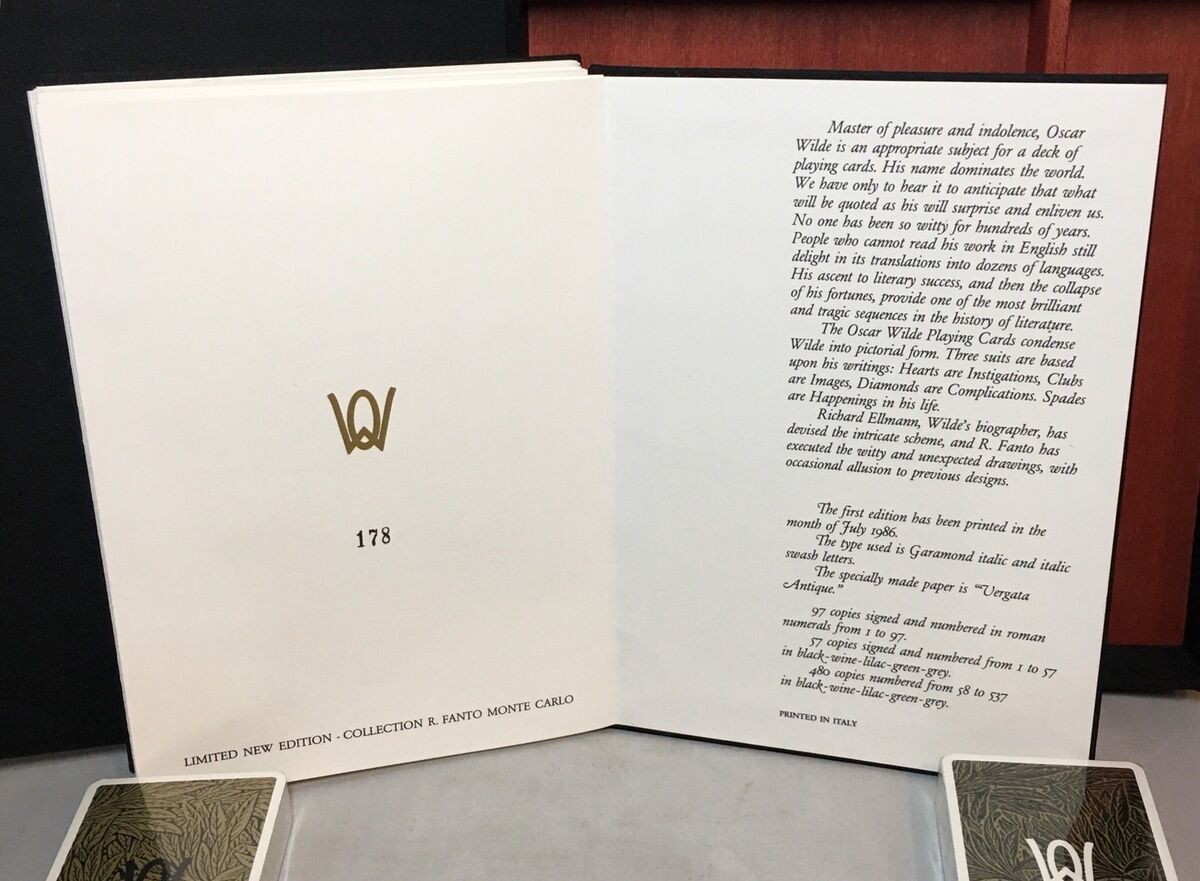The image presents an open booklet displayed on a reddish wooden surface. The left-hand page features a detailed layout, with a prominent O-W symbol at the top, followed by the number 178 beneath it. At the bottom of this page, in black text, it reads "Limited New Edition Collection, R. Fanto, Monte Carlo." The right-hand page contains extensive black text that provides context about the Oscar Wilde playing deck. It mentions that Richard Elman, Wilde's biographer, devised the intricate scheme while R. Fanto executed the witty and unexpected drawings with occasional references to previous designs. The booklet describes this special edition deck, first printed in July 1986, as a celebration of Oscar Wilde's legacy. Additionally, two box-like items, resembling playing card frames, are visible at the bottom of each page. These frames feature similar O-W symbols and decorative leaf designs against a light gray-green background on the left and a gray-trimmed black leaf design with a white symbol on the right.